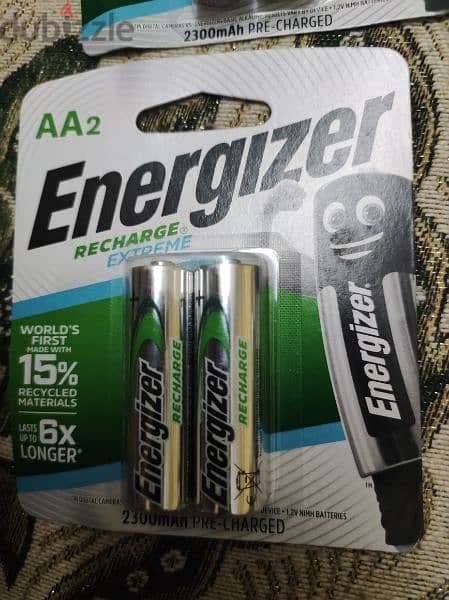This image showcases a pair of Energizer Recharge Extreme AA batteries. Prominently featuring the text "Energizer Recharge Extreme," these rechargeable batteries boast several impressive highlights: they are the world’s first batteries made with 15% recycled materials, designed to last up to six times longer with a capacity of 2300 mAh. The packaging and batteries themselves incorporate a color palette of green, blue, black, and brown, emphasizing the eco-friendly and high-performance nature of the product. No other details are present in the image.